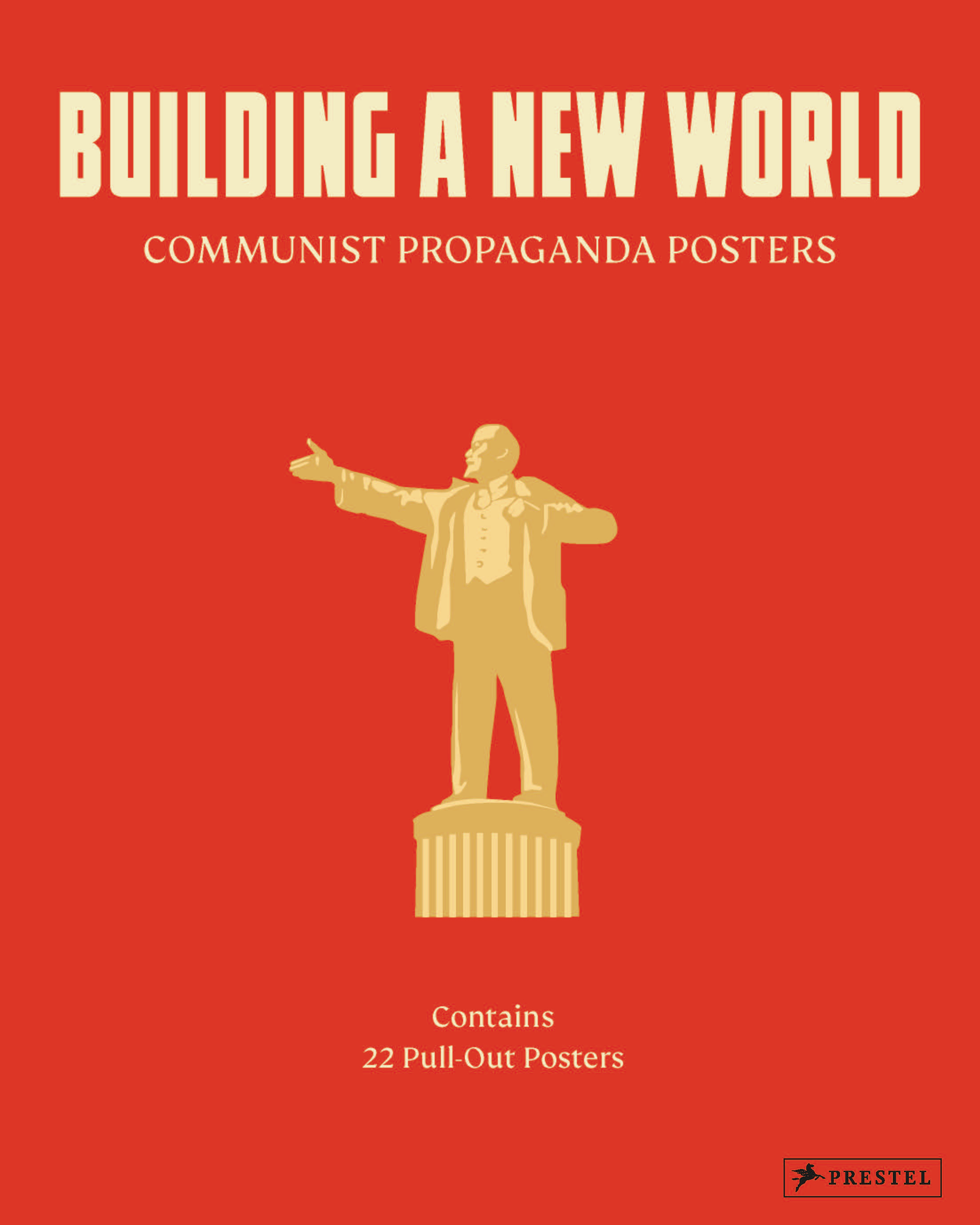The cover of this collector's book, titled "Building a New World" in bold, pale yellow capital letters against a bright red-orange background, prominently features a detailed thematic design. Below the main title, in slightly smaller capital letters, it states "Communist Propaganda Posters." Central to the cover is the gold and yellow figure of a man in a traditional Communist pose, standing on a small podium and extending his right arm outward. This man symbolizes propaganda figures and is illustrated in a stylized, statue-like manner. The cover also indicates that the book contains "22 Pull-Out Posters," highlighting its value for collectors of historical propaganda art. In the lower right corner, there is a small box with the publishing logo "Prestel," marked by a distinct rectangular border. This book likely showcases a curated collection of propaganda posters from various eras, such as the 1920s to the 1960s, offering insights into the visual history and iconography of communist movements.